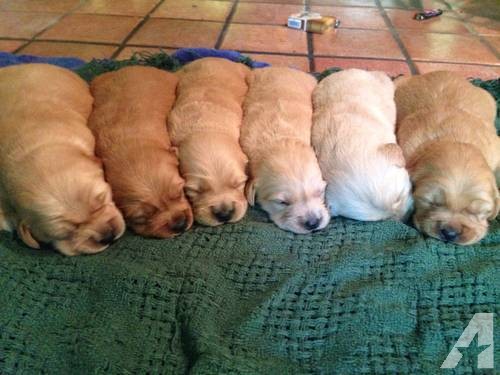This color photograph appears to be an informal snapshot, possibly seen on the news. The image prominently features a watermark in the lower right corner, a thick, stylized white letter "A" with the right side forming a straight vertical line and the left side slanting to the left. Inside the "A," a five-pointed star cutout is visible, with the star's top point creating the apex of the "A" and the side points forming the crossbar.

The scene shows six plump, young puppies of possibly Cocker Spaniel breed, arranged in a tight row across the middle of the image. They are all lying on a soft green blanket layered over a brown terracotta tiled floor, which is partially visible at the top of the image along with some unidentified objects.

The puppies, each in various shades of beige and brown, are cozily sleeping, with most facing the camera and their chins resting on the blanket. Their distinct colors range from light beige to almost caramel. The second puppy from the right is lighter than the others, with its head tucked sideways against a littermate, showing only the top of its head and hiding its nose. These young, sleepy puppies present a serene and heartwarming tableau.